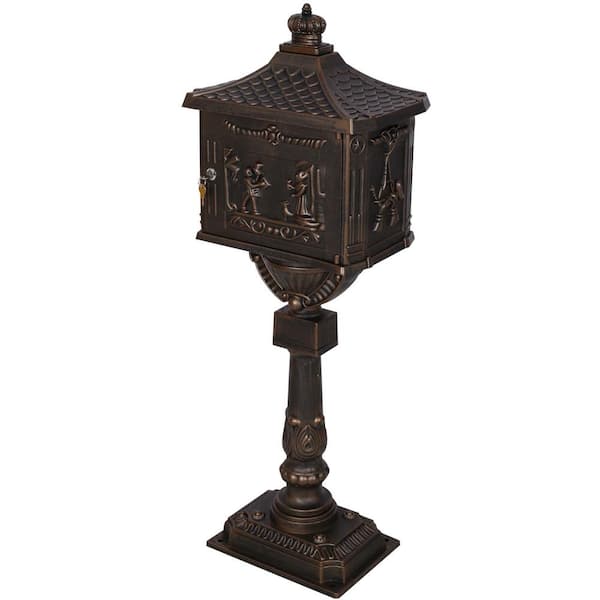The image depicts a small, ornate figurine set against a blank white background. The figurine, resembling a lockbox or ornamental container, is crafted from a dark bronze or brass-like metal. It features intricate carvings of ancient-looking figures and a distinctly decorative roof, reminiscent of thatched architecture, with sloping sides. A small key is visible, suggesting it can be locked and unlocked. The lockbox is mounted on a holder that begins with a rectangular base and transitions into a cylindrical, column-like structure adorned with decorative elements before merging with the box at the top. The rich, dark bronze finish and extensive ornamentation throughout give the piece an elegant, antiquated appearance, akin to a historical artifact or a meticulously crafted miniature sculpture.